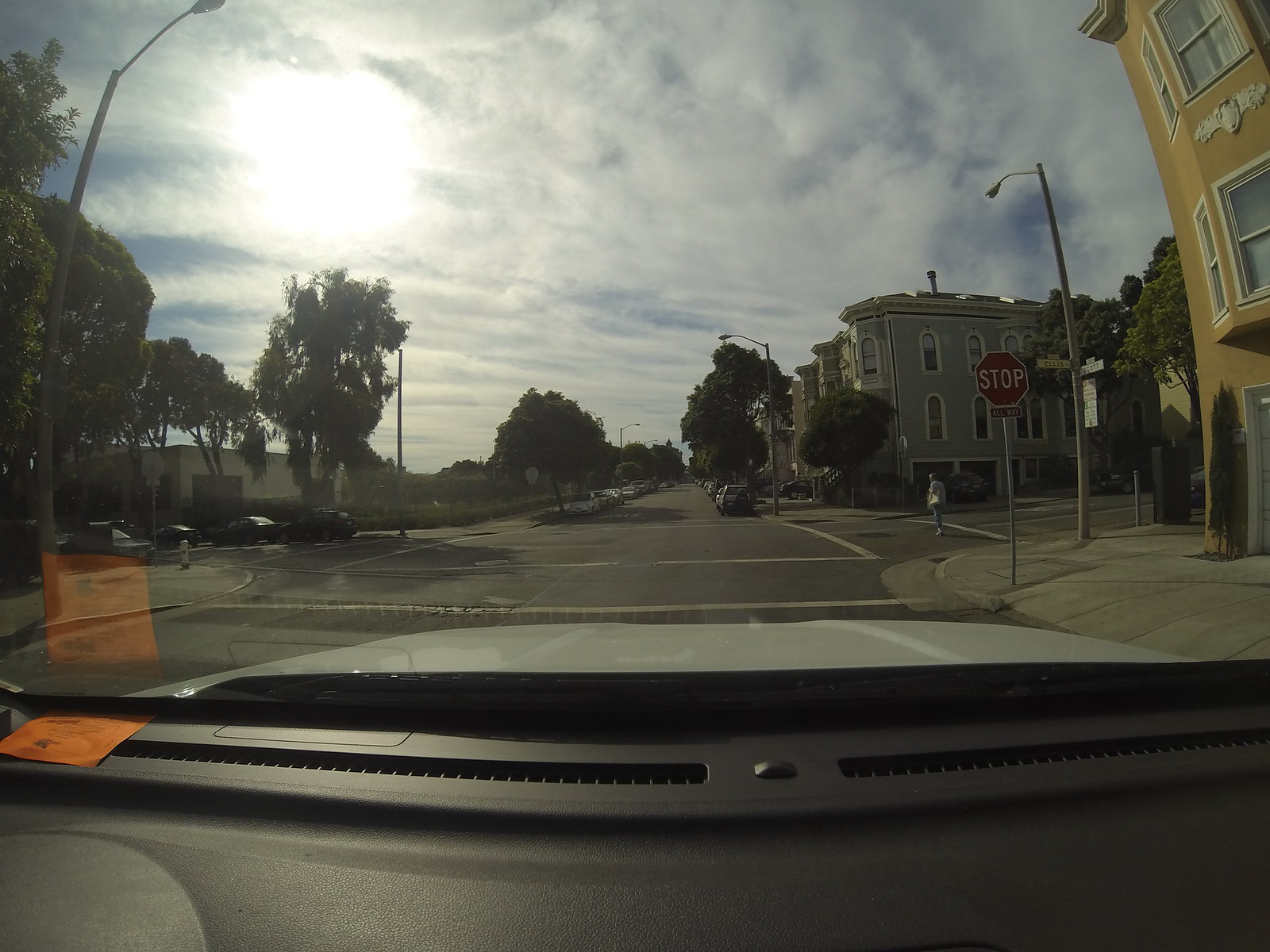In this image captured from a dash cam inside a silver vehicle with a black dashboard, we observe a picturesque street scene in a small town. The dashboard, featuring an orange parking permit to the far left, frames the view of a four-way intersection. To the immediate right of the vehicle is a stop sign, marking the center of this quaint urban area.

On the far right side of the image stands a brownstone building, characteristic of the town's architecture. Opposite this building, across the intersection, is another structure with a lighter, grayish-brown stone facade. This orderly street is further adorned with numerous tall, mature trees planted in a straight line, adding to the charm of the townscape.

At the intersection, we notice an individual crossing the street near the stop sign. The person, whose gender is indeterminate, is dressed in a white jacket and gray pants, traversing one of the crosswalks on a side street. The image captures not just the architectural details of the town but also a moment of daily life, painting a vivid picture of this serene small-town intersection.